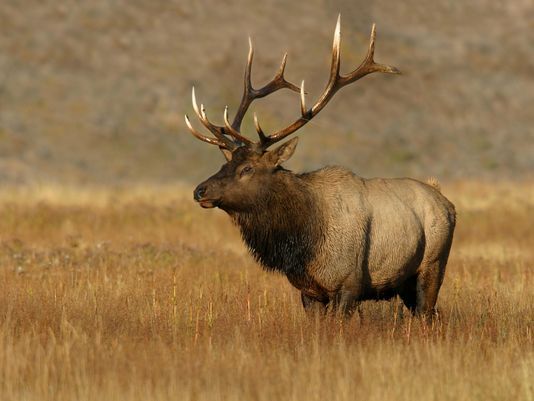This photo captures a solitary elk standing majestically in a field of tall, golden grass, which reaches up to its belly. The grass, appearing dry and unbroken by any other vegetation, spans across a backdrop of a yellowish-brown hillside, suggesting a Great Plains or prairie setting far removed from any civilization. The elk possesses a striking contrast in fur color, with a light tan body and a dark brown neck and head. Its grand antlers, featuring six pointed tines on each side, frame its head as it gazes pensively off to the viewer's left. The overall scene exudes an aura of serene wilderness and rugged natural beauty.